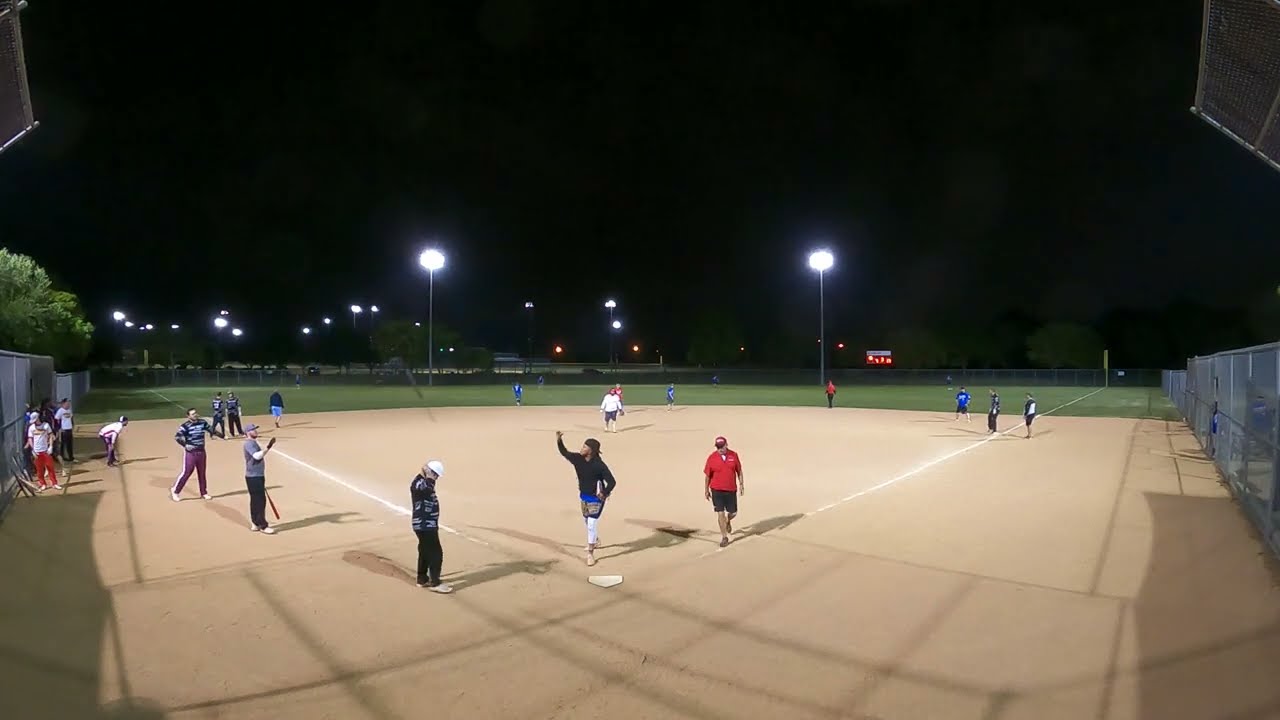In the image, a nighttime baseball game unfolds under bright illumination from numerous light poles surrounding the field. The well-maintained diamond showcases a stark contrast between the brown sand and the green grass that stretches into the outfield. Multiple players are poised at the bases, indicating an active game or possibly a training session. At home plate, a man in a black jacket waves to someone off to the left, while a coach dressed in a red shirt, matching red hat, and black shorts walks towards the viewer. In the outfield, players from the opposing team, distinguishable by their bright blue uniforms, are strategically positioned, anticipating a powerful hit. A pitcher in a white shirt stands ready on the mound, adding to the dynamic scene. Sporadically placed benches along the left side of the image and the fencing enclosing the diamond frame the bustling activity of the game.